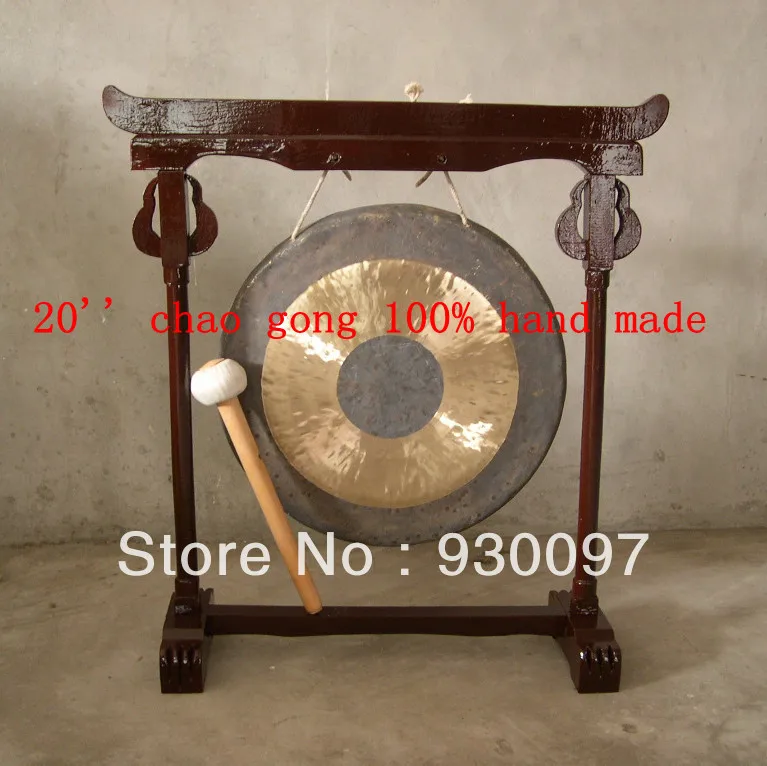The image depicts a large, round Chinese gong hanging from a sturdy, dark-stained wooden frame with intricate decorations that appear to be Asian-inspired. The frame, which rests on claw feet, supports the gong by two pieces of white rope. The foreground features a wooden club, designed for striking the gong, leaning against the frame; the club has a padded top that resembles a rolled-up sock to deaden the sound. The setup is situated on a concrete floor with a concrete wall serving as the backdrop. Prominently displayed over the image is red text stating "20 Chao Gong, 100% handmade," followed by white text that reads "Store No: 930097."